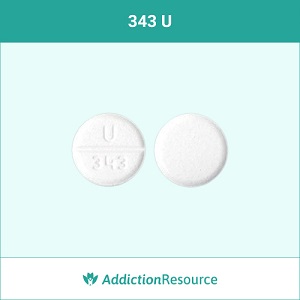The image features a square layout with a color scheme divided into two distinct sections. The top part of the image is a darker green shade, while the main part, which occupies most of the image, is a very light green. 

In the center of the light green area, two white pills are prominently displayed. The first pill, which is circular, has a score line down the middle, indicating it can be split. It features a large letter 'U' at the center and the number '343' on its bottom half. The second pill is also white but unmarked, except for the top, which has the imprint '343U'. 

At the very bottom of the image, the words "Addiction Resource" are written in green, with both 'A' and 'R' capitalized, forming 'AddictionResource' as a single word. A small icon of two people stands beside this text, overlaid with a green flower-like symbol. This careful arrangement and specific details suggest that the image is likely an informational graphic related to addiction treatment or awareness.